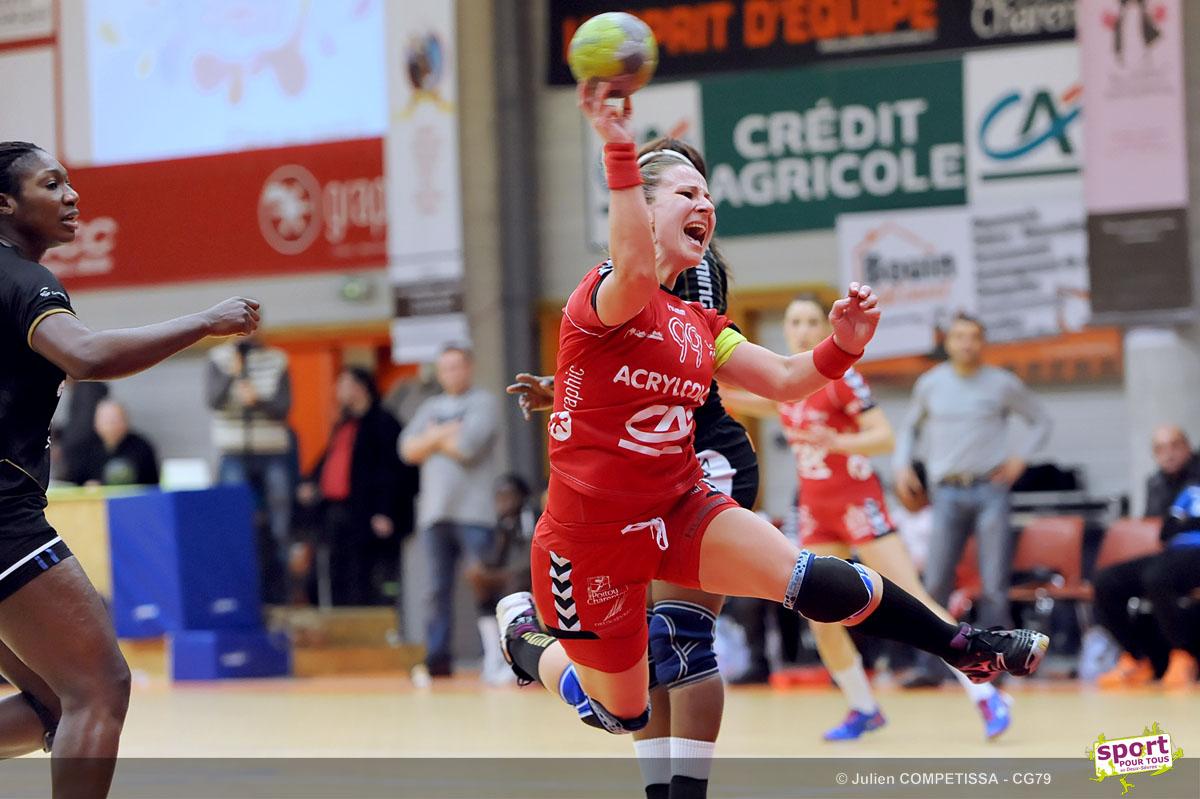This dynamic image captures a thrilling moment in a women's sporting event, likely a handball game. At the center of the photograph, a determined blonde woman in a red uniform, which includes red shorts and knee pads, is captured mid-air. Her left leg is bent behind her while her right leg is extended to the side with precision. She’s wearing tennis shoes and has a wristband on. Her left arm is raised, and her right arm is positioned to throw a small yellow and white ball, slightly larger than a softball. Her mouth is open, possibly shouting with the effort.

Directly behind her is a player in a black uniform with knee pads, partially obscured by the airborne woman, facing left. To the far left of the image, another player in a black uniform is bent slightly at the knees, with her hand extended in front of her, intently watching the action.

The background features a slightly blurry wall adorned with numerous banners and posters from sponsors, including Credit Agricole. The scene is set in a busy gymnasium with spectators lining the sidelines. A thin gray border runs along the bottom of the image, text on the right reading "Julian Competitza, CG79, Sportcore 2s, Pour Tous," with the word "Sport" clearly visible within an insignia of a little white card.